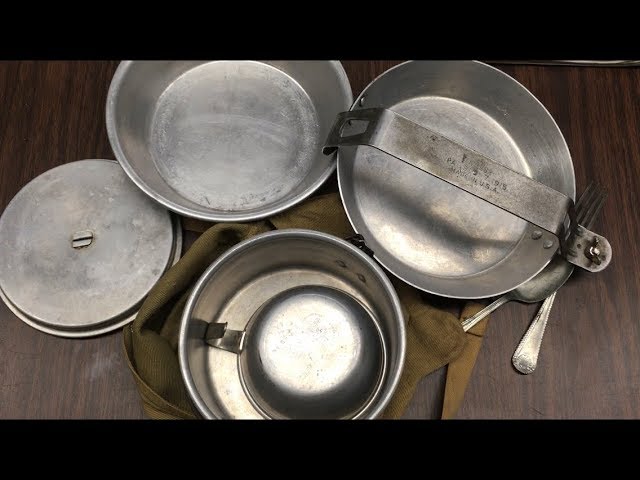This is an overhead photograph of a camping cookware kit arranged on a dark brown wooden surface with a grain pattern running vertically. The kit consists of shiny, silver, stainless steel or aluminum cookware, including two pans, a pot, a smaller saucepan turned upside down inside the pot, and a lid. An olive green cloth or bag is placed beneath the pot. On the right side of the composition, a spoon and fork are neatly placed, alongside a possible brown knife. One of the pans has a handle with a bar and wing nut system designed to lock the other pieces together. The entire setup gives the impression of a well-organized camping excursion. Two black bars frame the top and bottom of the image, emphasizing the central arrangement of the cookware.